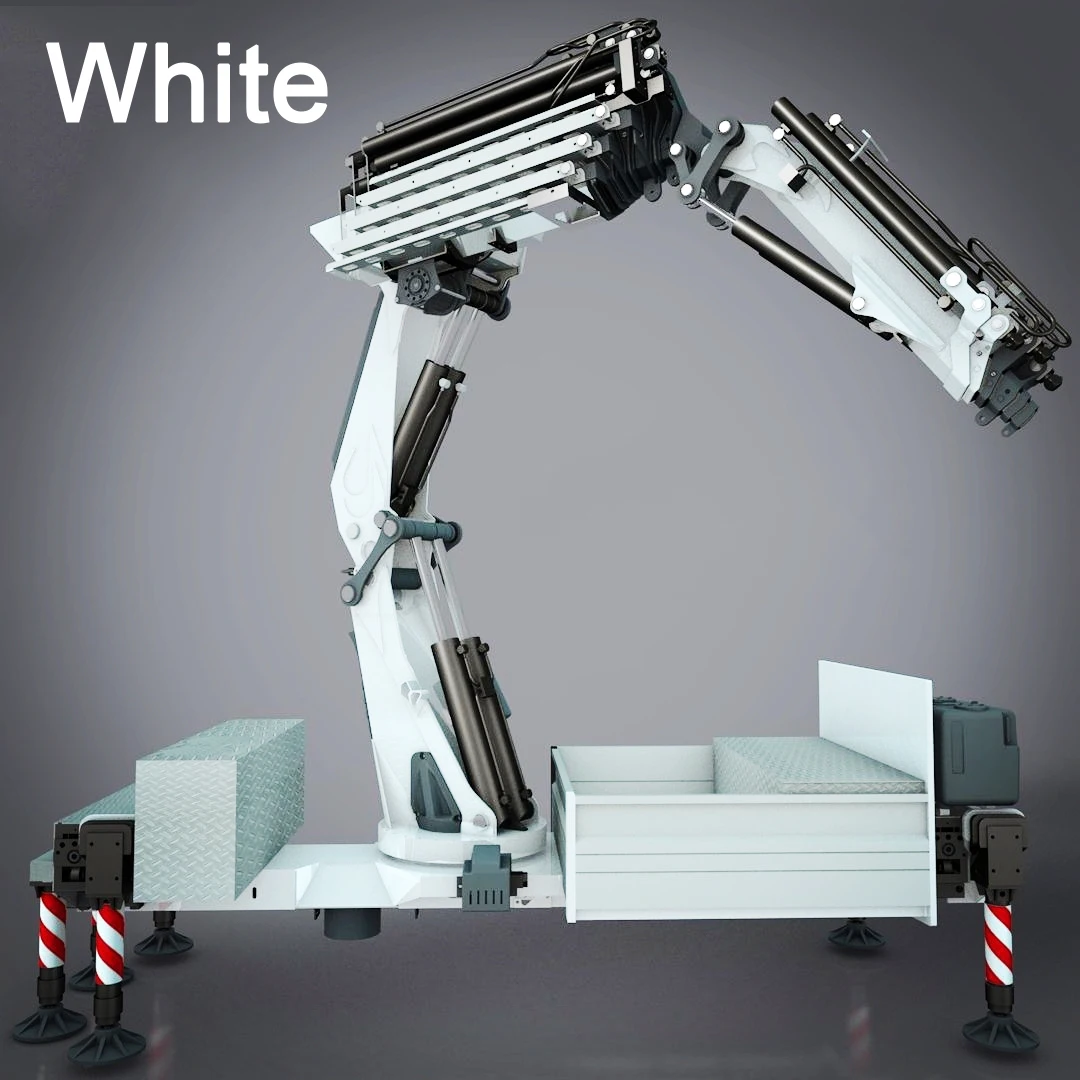This black and white industrial photograph showcases a sophisticated hydraulic manipulator, potentially part of a robot arm system, resting on a white platform. The platform is elevated about a foot off the gray ground, supported by four posts adorned with red and white candy stripe patterns and black bases. The manipulator is prominently white, with segments that include black pistons and steel bands. The arm, composed of four articulated segments, curves towards the right of the image. At the forward-most section, two small cameras appear to be mounted, likely for performing precise industrial tasks. The word "WHITE" is prominently displayed in white letters in the upper left-hand corner against a background that transitions from light gray at the center to darker gray at the edges. A toolbox sits nearby on the platform, hinting at the device's sophisticated, probably manual nature, as no extensive wiring or stepping motors are visible.